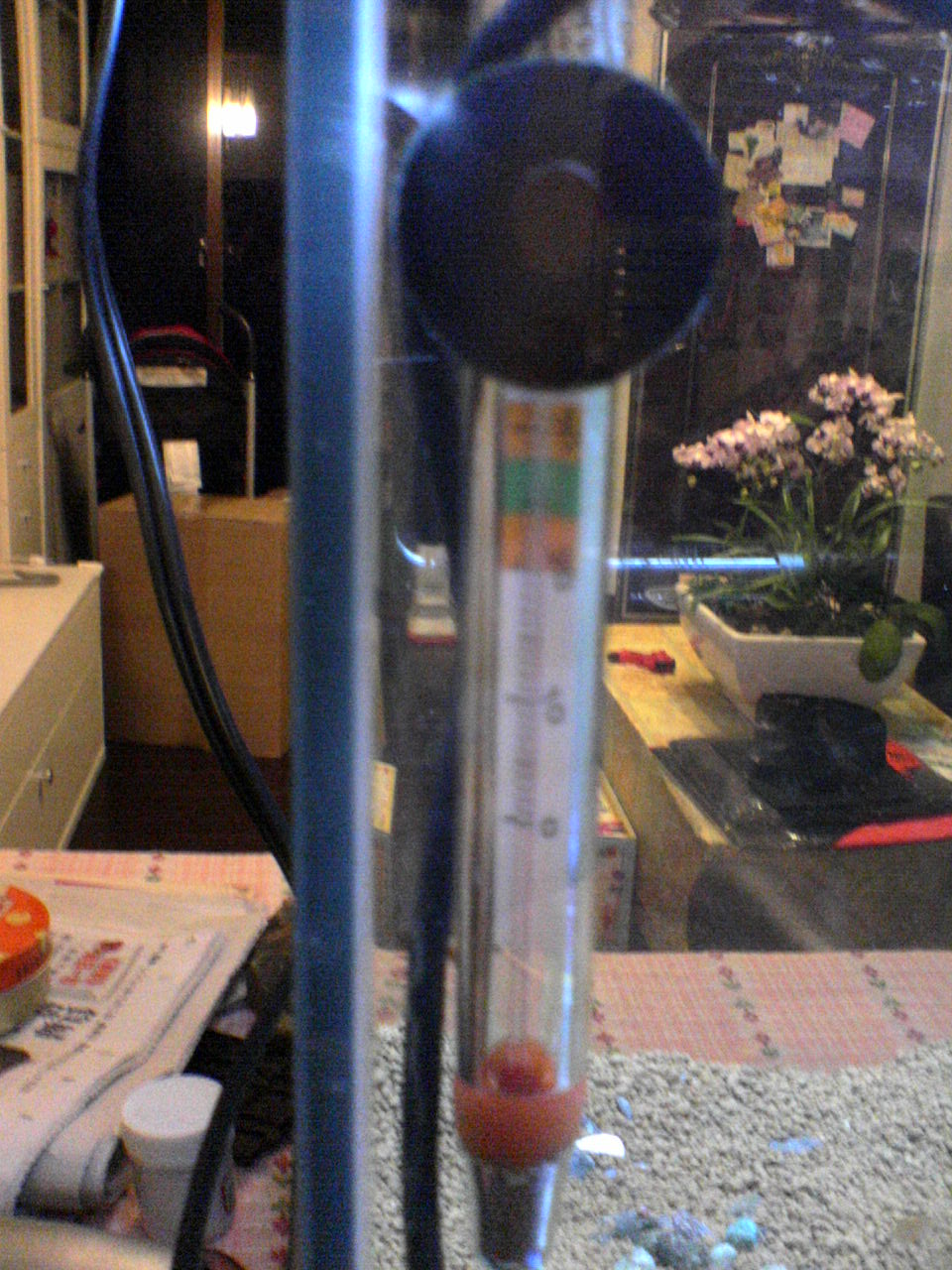In this grainy portrait image, the foreground prominently features a distinctive object resembling a pen. This object consists of a long, transparent tube marked with measurement notches, both small and large. Just below the tube, a red band is visible, followed by what appears to be a silver nib, possibly indicating it could be a thermometer. At the very top of the image, there's a black circular element, potentially a suction pad adhered to a window, providing a partial view through the glass.

A vertical metal strip descends from about two-thirds of the way over from the right, likely marking the edge of a mirror or window. The image's left side reveals a glimpse of what appears to be a book, placed in a room behind the foreground. Additionally, there is a small plastic tub at the front, alongside a cable extending above the frame's end. Scattered newspapers are also discernible.

In the background, on the left, stands a white cabinet with visible drawers, positioned in front of a brown set of drawers. To the right, behind the presumed window, is a surface adorned with a white porcelain planter overflowing with green leaves and pink-petaled flowers. A tall, rectangular black object, perhaps a fridge or door, looms in the rear, adding to the ambiguity of the setting. The image, overall, exudes the ambiguous atmosphere of either a living room or a doctor's surgery reception, making it challenging to pin down the exact location due to its grainy quality.